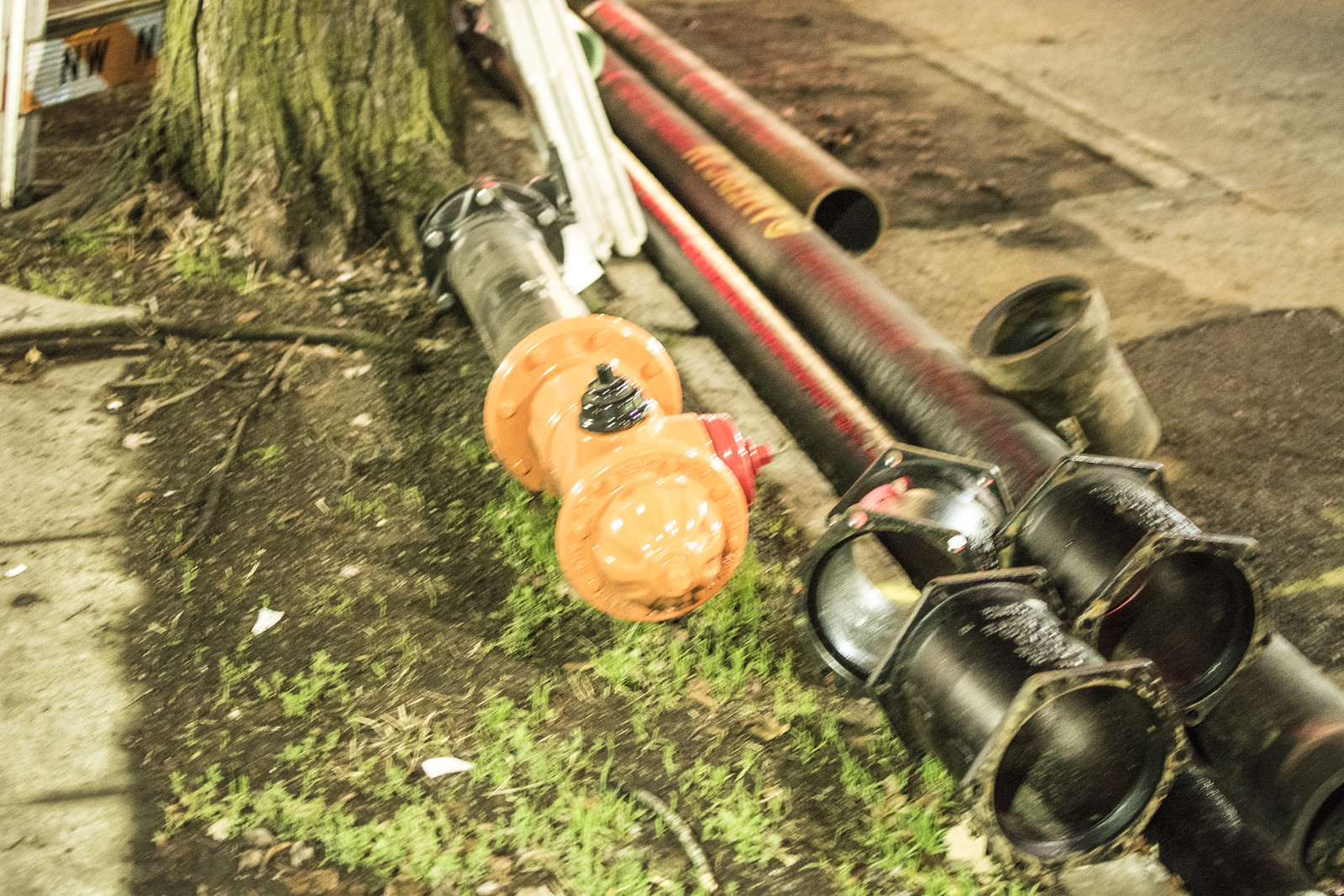This is an out-of-focus, messy streetscape photo featuring a collection of pipes and fittings scattered on a grassy area between a concrete sidewalk and a street. The sidewalk extends up the left side of the picture and contains two visible expansion cracks. A large tree, with rough bark covered in moss or algae, stands next to the sidewalk, with its base visible at the upper part of the image. Leaning against the tree is a red and white sawhorse with black lettering that reads "HW," though part of the text is obscured by the tree. The median between the sidewalk and the street is composed of black soil with some sparse vegetation and patches of dirt spilling onto the sidewalk. Various metal pipes with red markings and fittings, including orange and black ones, can be seen lying on the ground and near the curb. Additionally, there are short black pipe couplings with hexagonal bases and screw holes, and long lengths of pipe along the edge of the street. This scene suggests preparations for installing fire hydrants, evidenced by the detached glossy metal fire hydrant with a red main nozzle and black side nozzles, not yet installed but attached to a flanged pipe. The asphalt street is partially visible in the background, adding to the overall disorganized appearance of the setting.